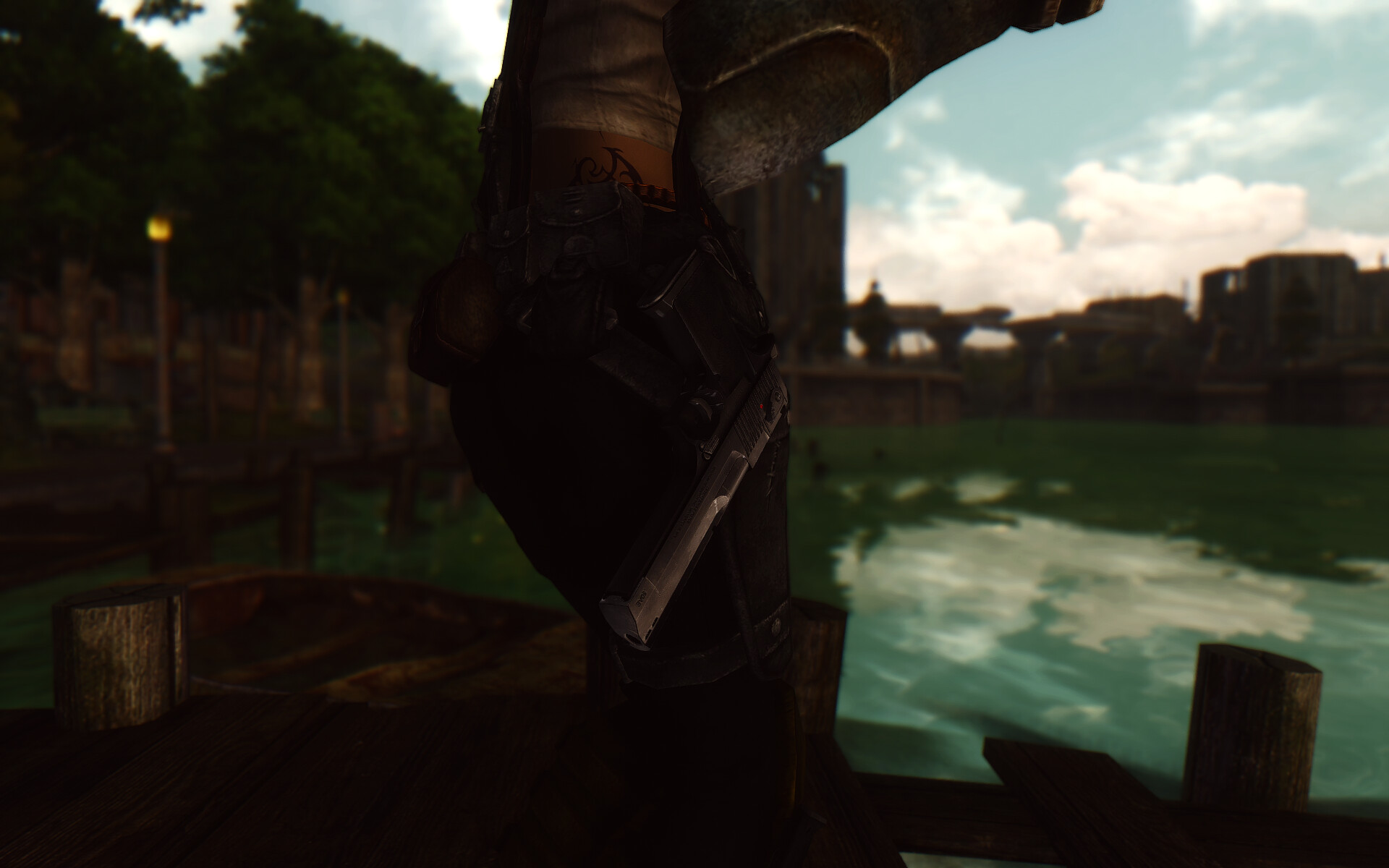The image is a very dark, shadowy, and slightly blurry outdoor scene, difficult to distinguish whether it is a photograph or a painting. The entire left side is immersed in shadows with indistinct silhouettes, save for a small golden-orange spot in the upper left corner and two bluish-white triangles that seem to either be holes or structures against the sky. The right side of the image seems to depict a body of water, possibly a canal or harbor, reflecting the cloudy sky above. The water has a greenish hue, indicative of its reflection. In the background, there might be silhouettes of buildings or possibly a bridge, shrouded in darkness and difficult to identify. Higher up, the sky is visible with blue tones and white, puffy clouds which might suggest overcast weather. The middle of the image hints at a central wooden object, potentially a glass or trophy, and features what appears to be older, dark concrete formations. Some trees are visible behind these concrete structures, adding to the outdoor ambiance, and no people or text are discernible in this indistinct, horizontal, and rectangular image.